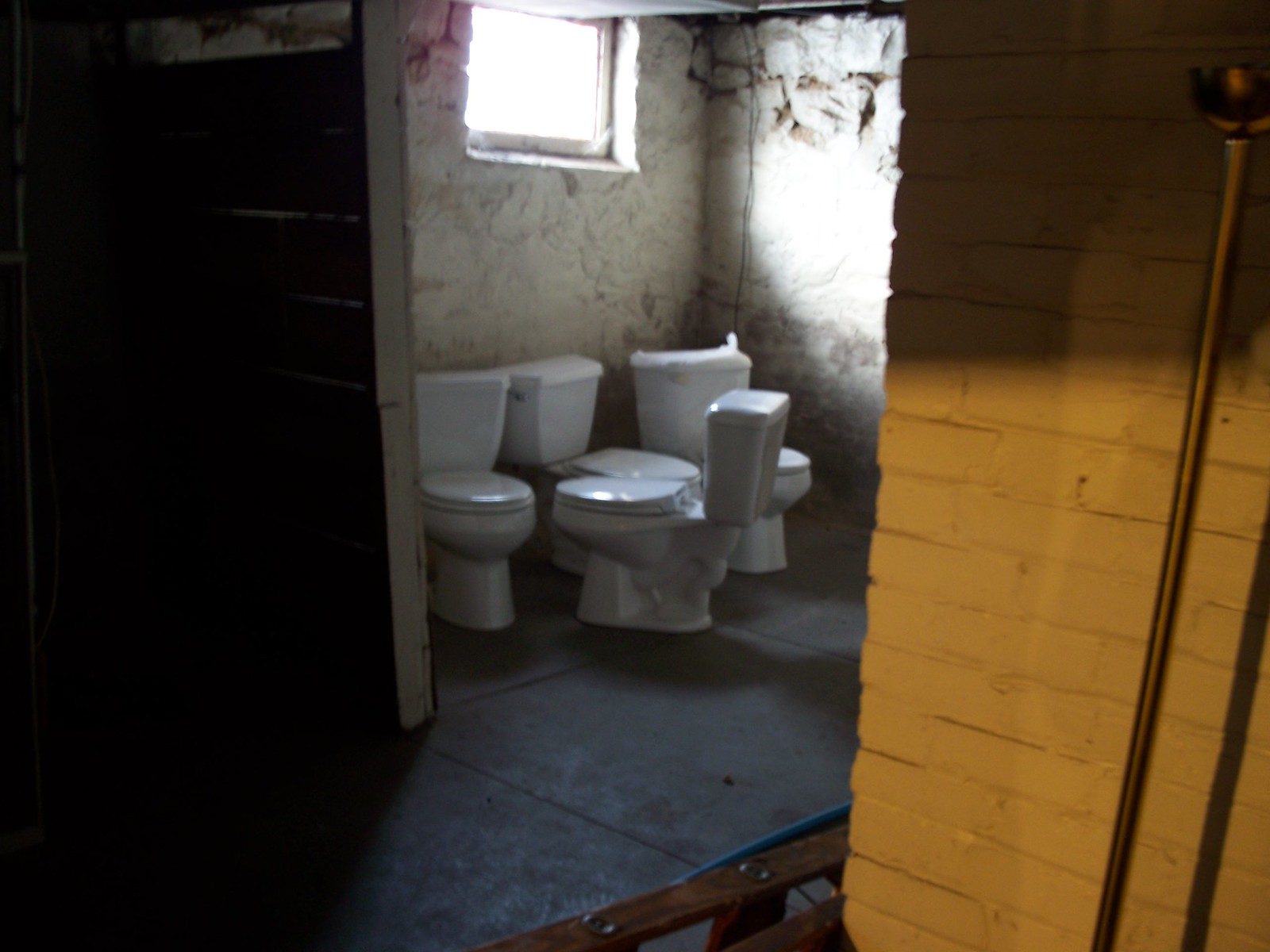This image captures an eerie and dimly lit basement, possibly abandoned or unfinished, characterized by its crumbling, white-painted brick walls and dank atmosphere. At the center of this bleak scene are four white porcelain toilets, clearly not in use and seemingly stored haphazardly in the small, grimy space. Three of the toilets face outward towards the viewer, while the fourth is positioned to face the others directly, creating an odd congregation. The floor, likely concrete, is covered with a mix of dirt and scattered objects, including what appears to be a ladder. The room is partially illuminated by a single, small window that casts a diagonal beam of light, enhancing the sense of neglect. Copper pipes and some sort of brass structure are visible along one of the walls, adding to the unfinished industrial look. The overall setting gives off a strong impression of a storage area within a neglected basement, with an unsettling, abandoned feel.